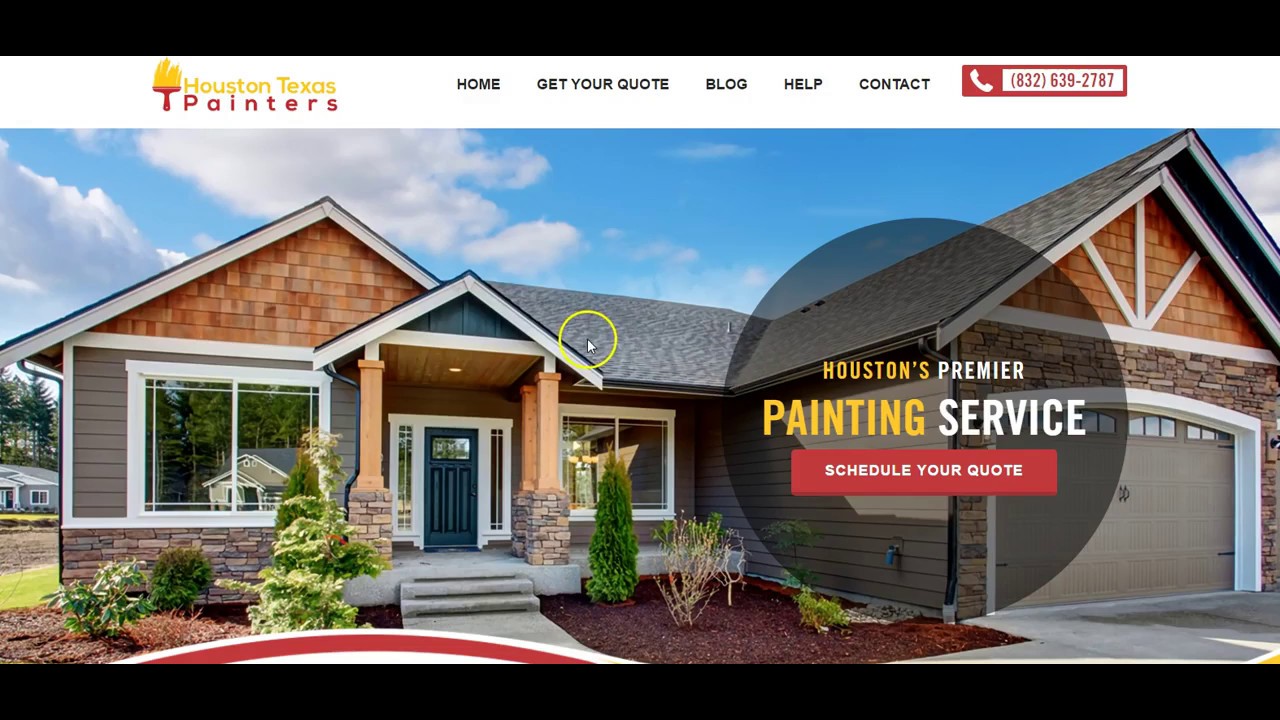At the top of the image, there is a black bar displaying an icon for "Houston, Texas Painters." Below this bar, you'll find the navigation options: Home, Get Your Quote, Blog, Help, and Contact. A red bar features a phone icon and a contact number, (832) 609-2787. The sky is blue with a few white clouds.

The main part of the image showcases a house with a detailed facade. There are brown panels, white, and gray shades, and a yellow circular design. The house features pillars, a door, and surrounding lights. To the left and right, there are planted areas with green trees and soil, accentuated by wood panels and cement walkways. On the right side of the house, there is a brown garage with a white border and a cement driveway, which has visible oil stains.

The top section of the house includes additional brown paneling. On the left side, there's a faucet, and the lower part of the wall features decorative stones. In the background, another house with gray walls and additional trees can be seen. The sky overhead is a clear blue.

A prominent circular logo in the center of the image reads "Houston's Premier Painting Service." Below it, a red rectangle with white text instructs viewers to "Schedule Your Quote."